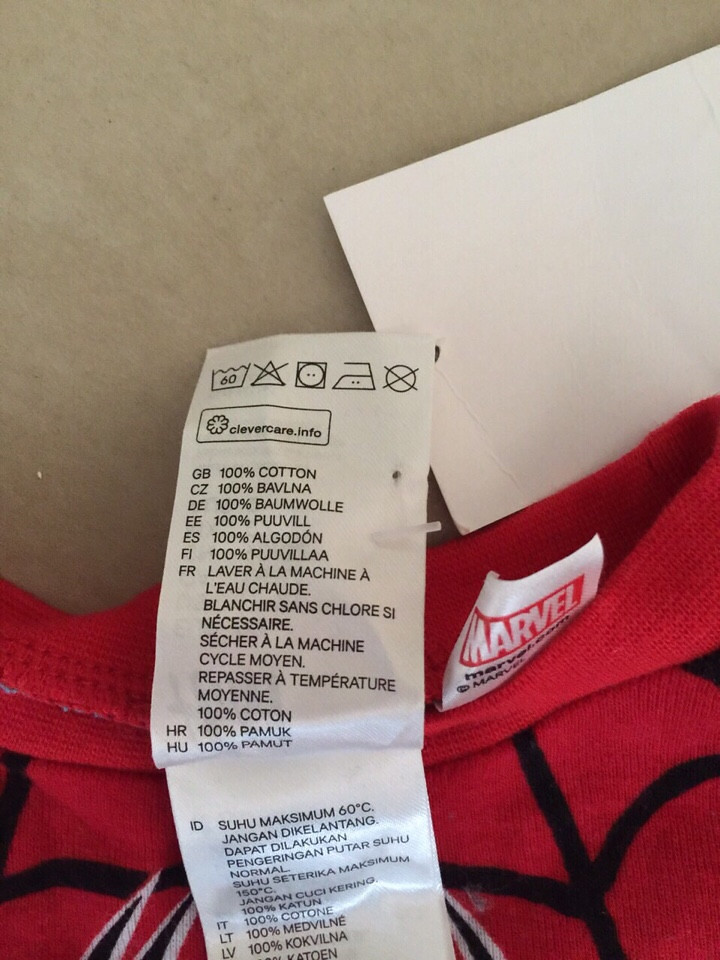In this vertical rectangular image, we are presented with an almost overhead, aerial-like perspective. The upper portion of the background is a tan beige color with subtle streaks, giving it a slightly varied appearance, rather than a flat, uniform look. Emerging from the right side of the image is a white piece of paper. This paper appears slightly wrinkled and creased, adding an element of texture. Dominating the center of the image is a bright red Marvel T-shirt featuring black lines, potentially indicative of a Spider-Man design or claw marks, although only a portion of the neckline area is visible, making it difficult to discern the exact pattern. The T-shirt's white tag is lifted, revealing crucial information printed on it, notably stating that the shirt is made of 100% cotton. The tag also contains additional details in multiple languages, providing further garment care and information.